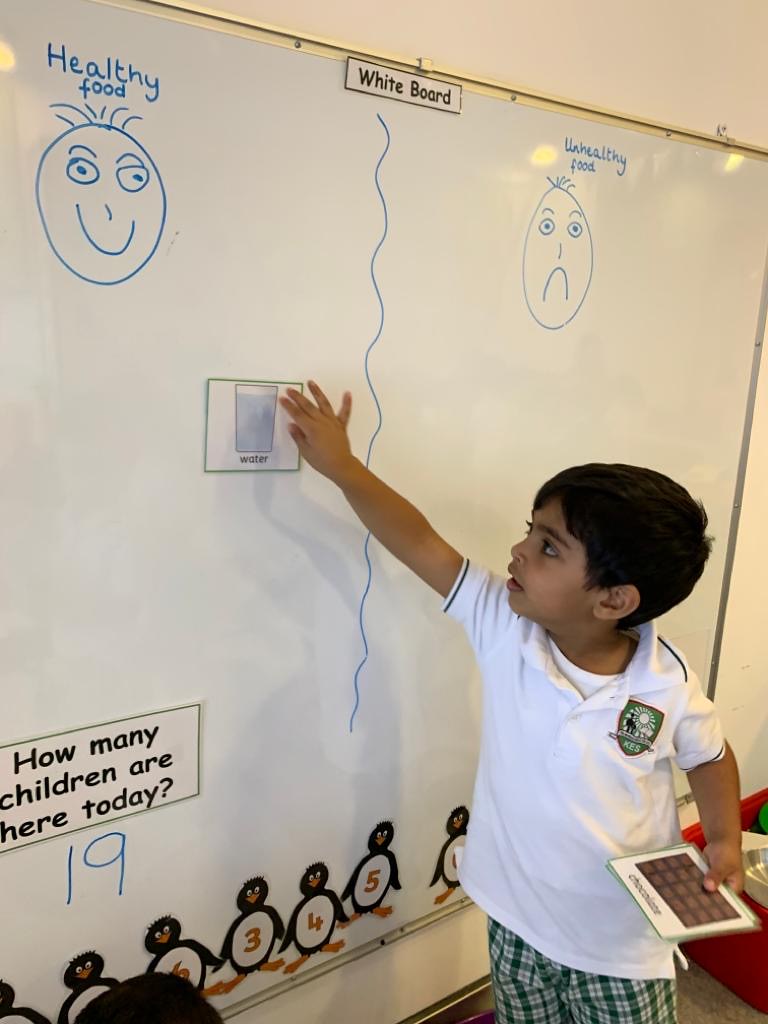In this photograph, a young boy stands attentively at a classroom whiteboard, actively participating in a lesson. The whiteboard, divided into two sections by a vertical line, categorizes foods into "healthy" and "unhealthy." The healthy side, identified by a smiley face with a few strands of hair drawn above it, includes the label "Healthy Food," while the unhealthy side features a frowny face and is labeled "Unhealthy Food." 

The boy is keenly placing a magnetic card depicting a glass of water into the designated healthy section. In his other hand, he holds a card with an image of chocolate, seemingly contemplating where to position it. Dressed neatly in a white collared shirt and green-and-blue checkered shorts, he epitomizes the engaged and well-dressed student. 

Above the whiteboard, a small sign with the word "whiteboard" in black text is affixed at the top center. Off to the left side of the board, "How many children are here today?" is written, with the number "19" marked in blue beneath it, reflecting the day's attendance.